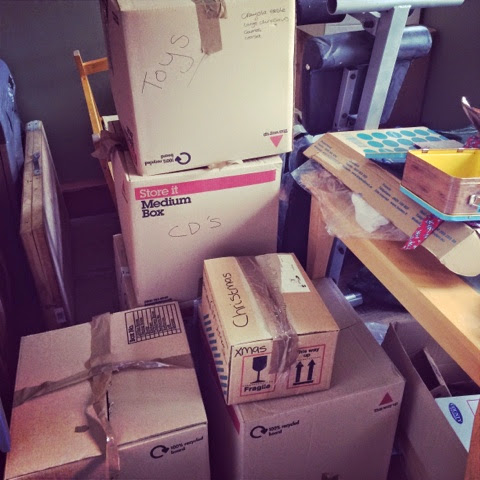The image depicts a cluttered room filled with various brown moving boxes and a wooden work table towards the right side. In the center of the picture, two medium-sized boxes are stacked on top of each other; the bottom box is labeled "store it, medium box" with "CDs" handwritten on it, while the top box has "toys" written in black marker on the side. In front of this stack are two more boxes on the ground. The box on the left is partially covered with packaging tape, and the right box has a smaller rectangular box on top, labeled "Christmas" in marker and also taped shut. To the right of this setup, the wooden work table is cluttered with various items including an open long box, a small metal container with a yellow interior sitting on a blue lid, and a stack of large circular blue objects. The background is relatively sparse, revealing parts of a dark wall and a baseboard, with unclear details of possible additional objects like a chair and a shelved unit. The overall scene is one of disorganization, with boxes both on the floor and seemingly placed on or around furniture.